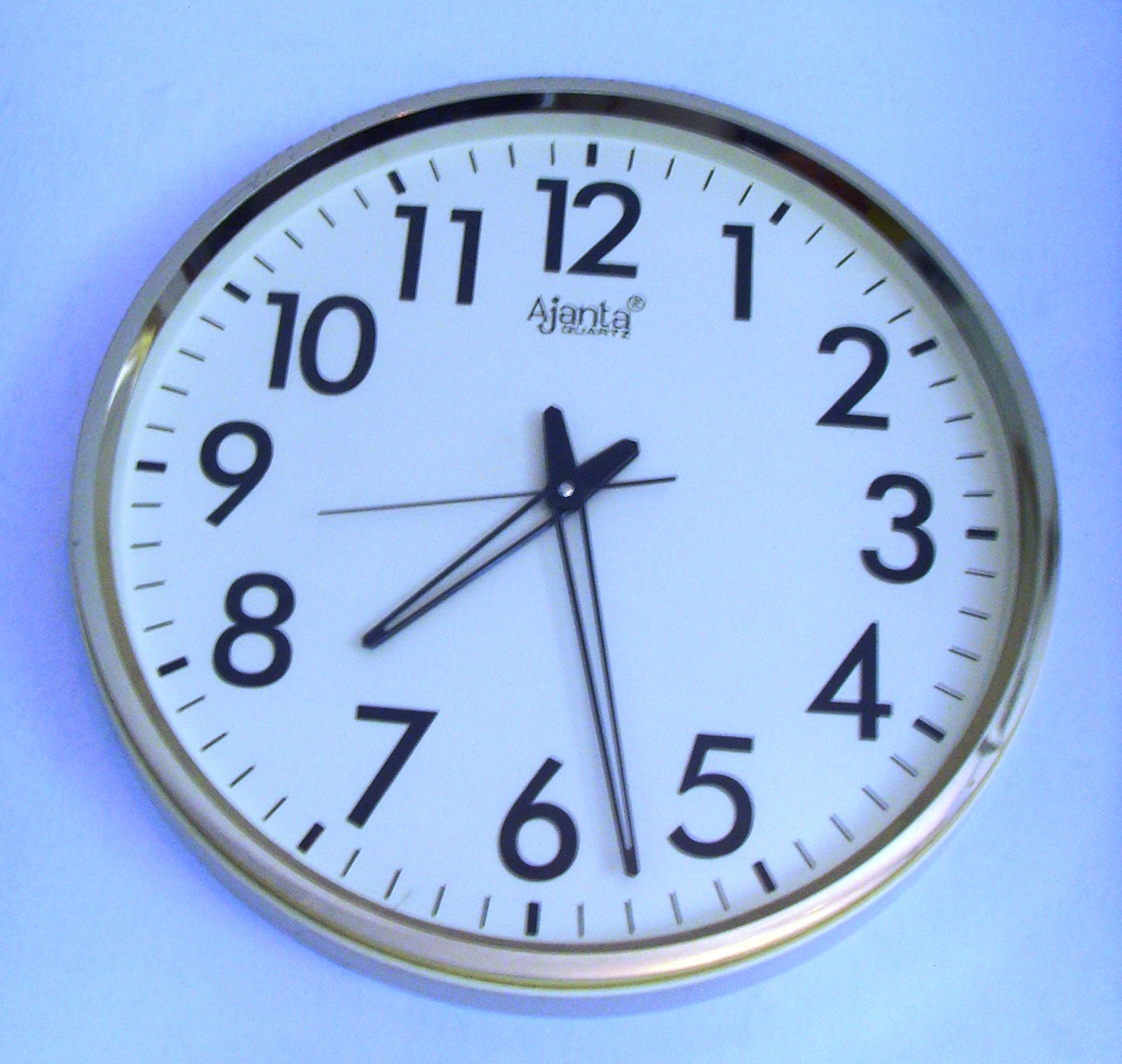This image showcases a clock set against a light blue wall, which gradually darkens towards the top. The clock features a modern design with a silver metal frame and a brownish inner lining. Its face is white with big bold black numbers (1 through 12) and black notches for minute markers. Above the 12, the brand name "Ajanta" is prominently displayed with a circled trademark symbol, and "Quartz" is inscribed below it. The clock hands have a distinctive design: black outlines with hollow interiors, ending in sharper points. The clock shows a time of approximately 7:28 and 43 seconds, with a thin, short second hand just below the 9 and nearing the 12. The clock, despite its detailed features, serves a basic functional purpose.